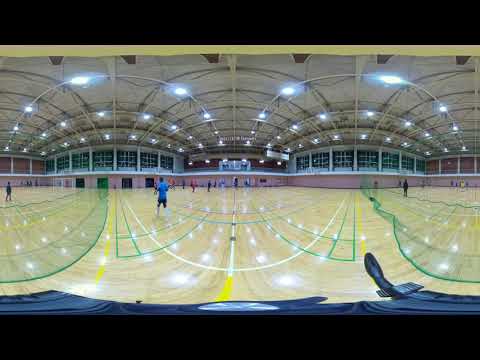The image depicts a panoramic view of a gymnasium, likely a basketball court, divided into three distorted and curved sections, with the central section appearing as though viewed through a bubble. The court floor is light brown with green and blue lines marked on it, reflecting the white, linear lights from the ceiling. There are several visually prominent features: a domed roof with arced lighting arrangements, rows of white and gray bars, and a tiled white ceiling interspersed with windows. 

In the central section, a gentleman wearing a blue shirt and black shorts stands to the left, while other figures clad in dark attire can be seen in the background. On the right and left sections, similar scenes unfold with slight variations in angles but consistent elements like the light brown floor, ceiling lights, and background walls. The upper walls exhibit white surfaces punctuated with windows, while the lower walls are pink with a distinct white ledge separating the two levels, giving the appearance of a two-story structure. In the far background of all sections are vast glass windows offering a potential view of the cityscape, suggesting a spacious, multi-use indoor sports facility.